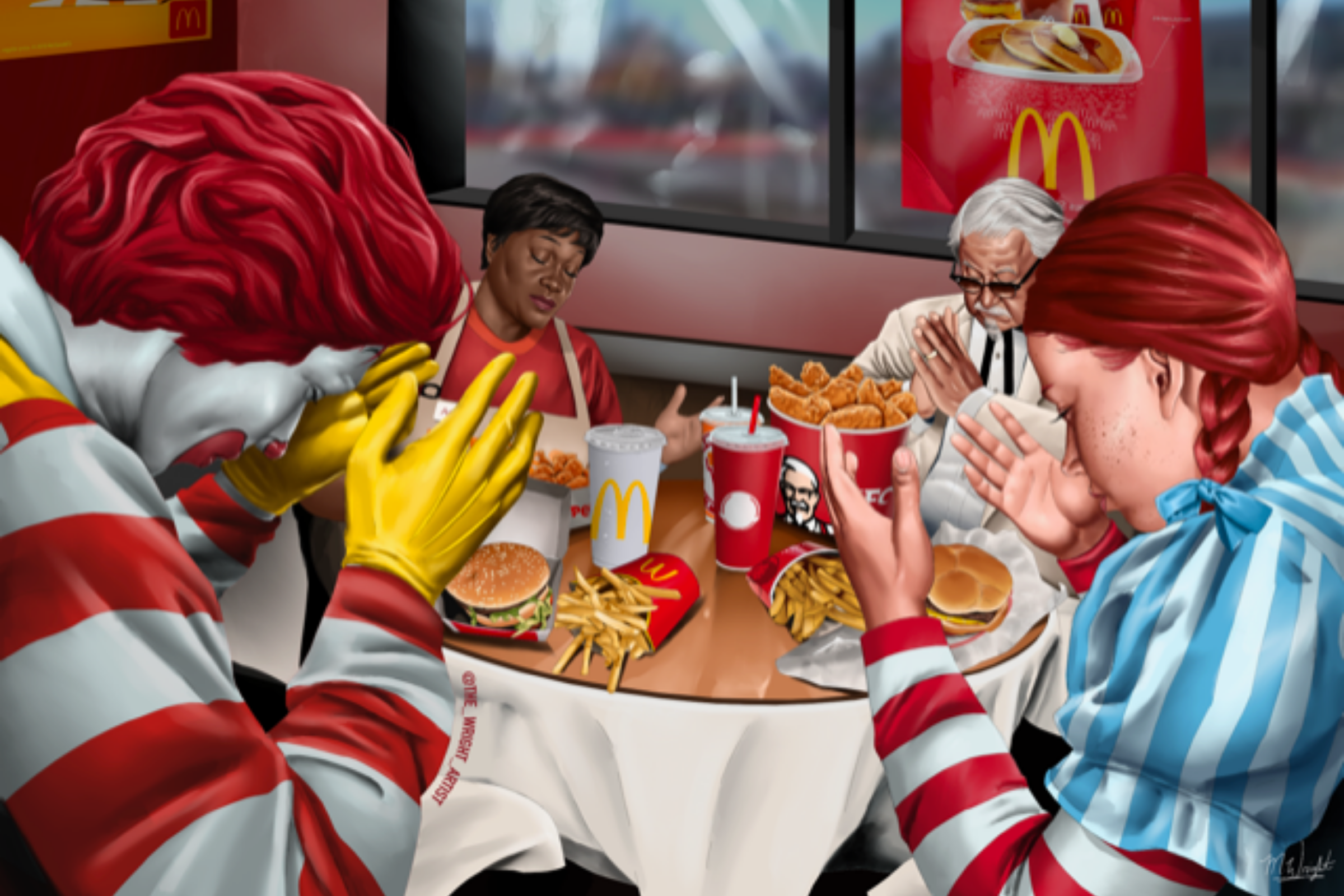This is a detailed, computer-generated animated restaurant poster featuring mascots from various fast-food chains, all gathered around a round dinner table. The table itself has a white tablecloth underneath a glass circle, and all characters have items from their respective restaurants in front of them. Starting from the left, there's Ronald McDonald from McDonald's, easily recognized by his red hair, yellow gloves, and red and white striped shirt, with a burger and fries in front of him, his hands folded as if in prayer. Next to him sits the African-American woman from the Popeyes commercials, wearing an apron, with Popeyes food before her. Continuing around the table, we see Colonel Sanders from KFC, identifiable by his iconic white suit and black string tie, holding his hands together in front of a bucket of chicken. To his right is Wendy from Wendy's, with her signature red braided hair, positioned with her hands out in front of her, also appearing to pray, a sandwich and fries in front of her. They all have drinks by their meals. The background reveals a McDonald's setting, evidenced by a McDonald's sign and a poster for McDonald's breakfast visible through the blurry, red-hued windows. A faint, indecipherable signature appears at the bottom right of the image, completing this surreal assembly of fast-food icons.